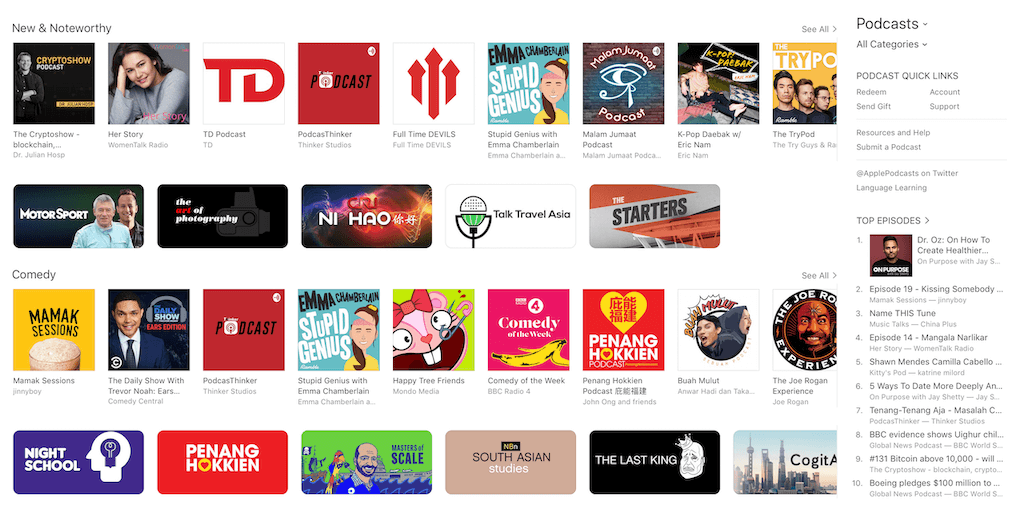Screenshot of a Podcast Directory Interface

The image showcases a screenshot of a podcast directory website, featuring an organized layout of various podcast cover arts, categorized under different sections. Notably, the first category is labeled "New and Noteworthy," highlighting several prominent podcasts such as Crypto Show Blockchain, Her Story, TD Podcast, Podcast Thinker, Full-Time Devils, Stupid Genius with Emma Chamberlain, Madam Jamai Podcast, K-pop, The Tripod, Motorsports, The Art of Photography, Talk Travel Asia, The Starters, CRI and How, and numerous other series.

The cover arts in this section boast a wide array of background colors, including gold, white, gray, red, teal, black, green, pink, and purple. Among them, there's even one with a city skyline background, adding a distinct visual element. Various genres are represented, such as comedy, with titles like Mom X Sessions, The Daily Show with Trevor Noah, Happy Tree Friends, Comedy of the Week, Pyeongho Com Podcast, Bum Mullet, The Joe Rogan Experience, and Night School. The listing also includes discussions on South Asian Studies and unique entries like The Last King.

On the right side of the screen, there are options presented in black text against a white background, labeled "Podcast: All Categories." Beneath this heading, quick links are provided for functions such as "Redeem," "Send Gift," "Account Support," "Resources and Help," "Submit a Podcast," alongside a Twitter link. Additionally, themed sections like "Language Learning" and "Top Episodes" are visible, with the latter featuring a top 10 list of popular podcast episodes.